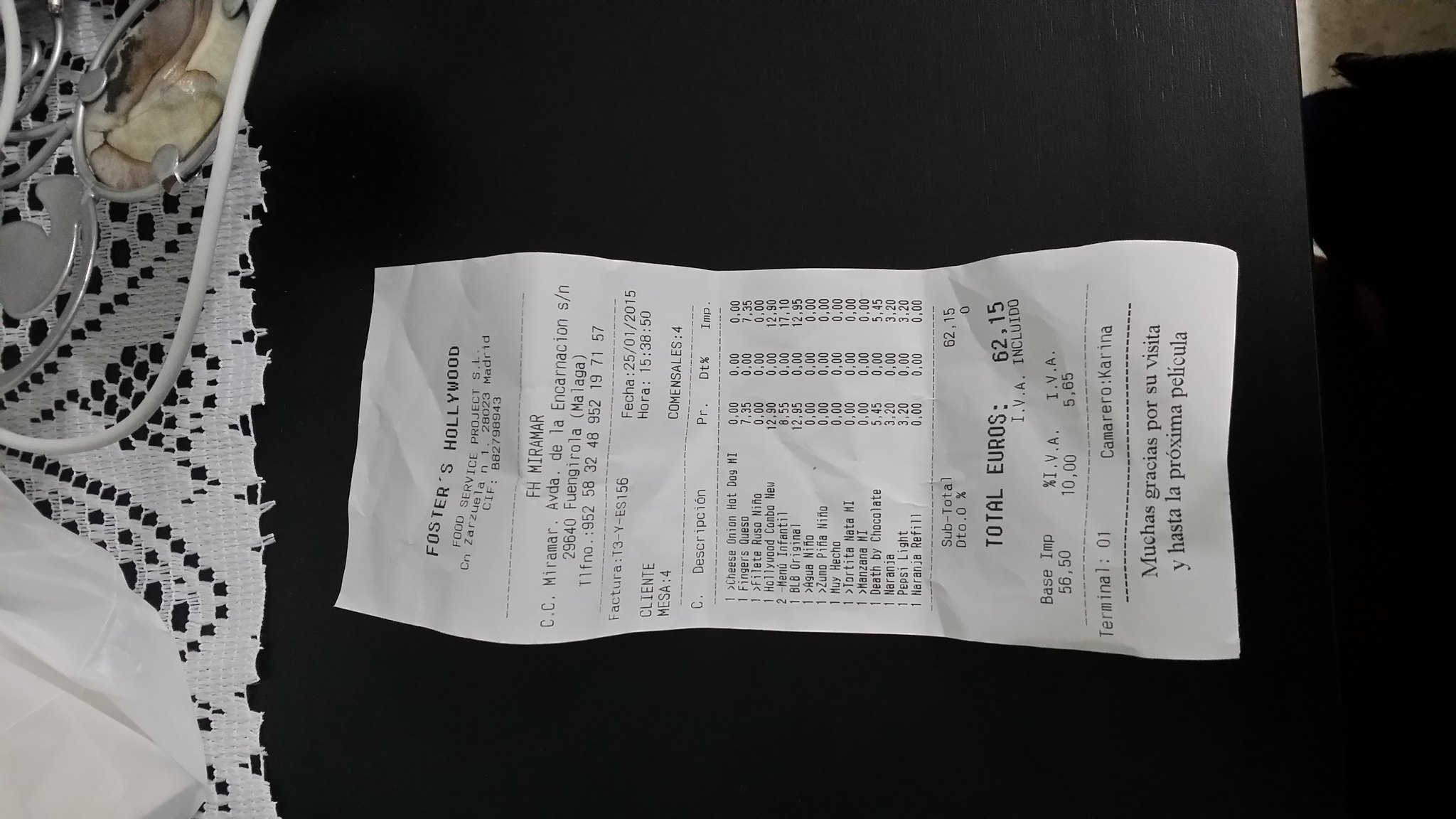A close-up shot captures a detailed view of a receipt from Foster's Hollywood restaurant, placed on a dark wooden table beside a lace doily. The receipt, amounting to 62 euros, lists items such as a cheese onion hot dog, fingers queso, and the Hollywood combo new. The bilingual formatting of the receipt—with text in both English and Spanish—suggests a location in Spain, further supported by the message "Muchas gracias por su visita y hasta la próxima película" printed on it, indicating a courteous thank you and an invitation for a return visit.